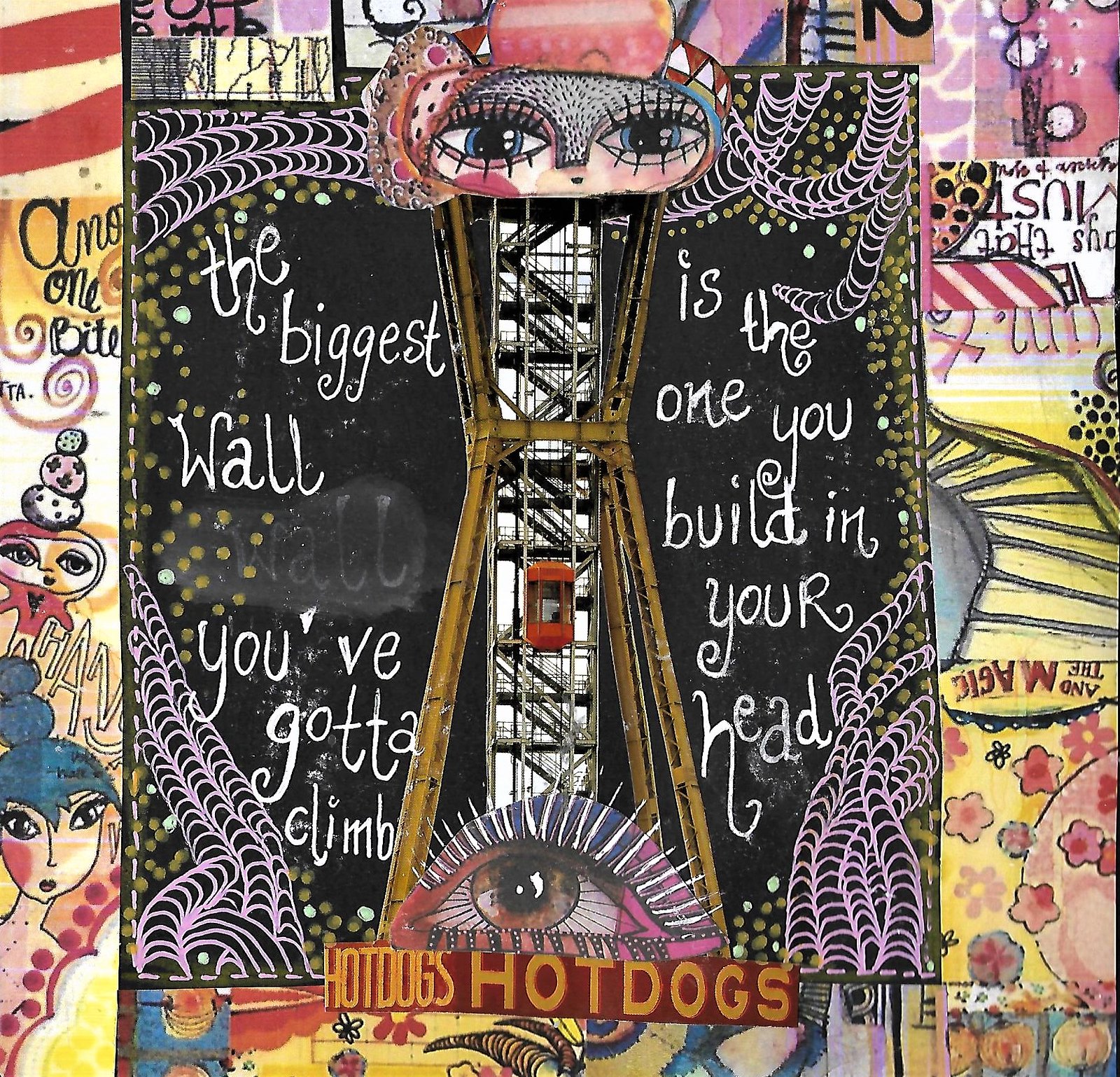This detailed mural, painted on the side of a building, features a vibrant and eclectic mix of elements that cohesively form a striking visual narrative. At the mural's focal point stands an artistic representation of the Eiffel Tower, complete with a centrally ascending red elevator. The tower is framed within an intricate yellow hourglass structure, reminiscent of bamboo. Cartoonish eyes peer out from the top of the tower, giving it a whimsical face-like appearance. Beneath the tower is a vividly illustrated eyeball, adorned with eyelashes and makeup, gazing upwards. Directly below this, a red sign with yellow lettering prominently advertises "hot dogs" twice.

The mural's background is a tapestry of diverse colors and patterns, ranging from animated figures to abstract designs, including roads, railways, bridges, and spiral motifs. The entire composition is bordered with multicolored sections, featuring a red and white striped area in the upper left, accompanied by the text "Ano One Bite" on a yellow background.

A poignant message is inscribed in white chalk-like print on the black surfaces flanking the central image: "The biggest wall you've got to climb is the one you build in your head." This phrase is partially repeated and edited, adding a layer of depth and reflection. Among the figures depicted, a woman directly engages the viewer by looking straight into the camera, while a boy whimsically balances three balls on his head. This mural is not just a visual feast but also a profound commentary on personal barriers and potential.